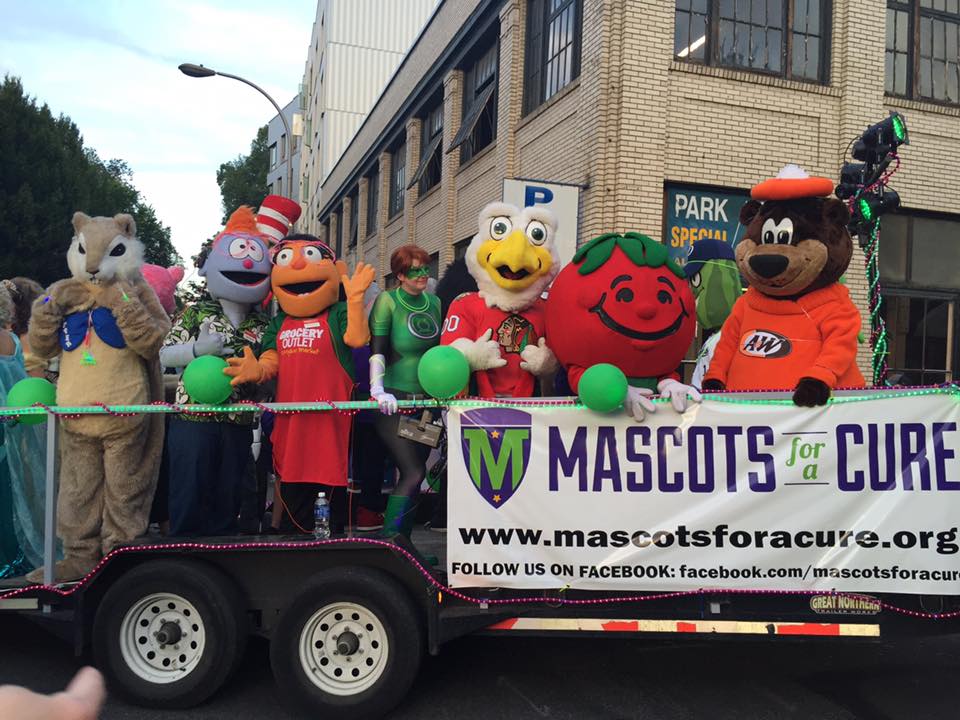In this full-color, square photograph taken during a daytime parade with natural light, we see a vibrant float from "Mascots for a Cure" moving through a street framed by multiple-story brick buildings. The flatbed trailer is adorned with a prominent banner that reads "Mascots for a Cure, www.mascotsforacure.org, Follow us on Facebook." The float is bustling with a diverse array of mascots: on the far right stands an A&W bear mascot clad in an orange outfit and hat, next to a tomato character. The middle features a duck mascot in a red jersey giving a thumbs-up. On the left side, there's an assortment of characters including a teen mascot, a Native American figure, and a squirrel with a white face and brown body with something blue on its chest. The background reveals a brick building with multiple stories and windows. The sky, visible in the upper left corner, shows patches of blue with white clouds on what appears to be a partly sunny day.